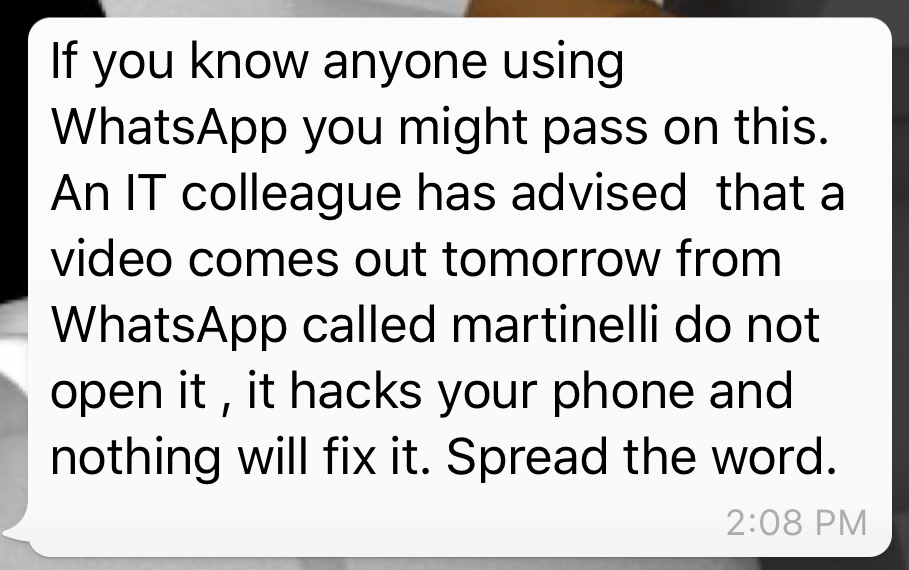The image depicts a clear, zoomed-in picture of a text message. The message, displayed in black text on a white background, reads: "If you know anyone using WhatsApp, you might pass this on. An IT colleague has advised that a video comes out tomorrow from WhatsApp called Martinelli. Do not open it. It hacks your phone and nothing will fix it. Spread the word." The time stamp 2:08 PM is prominently shown at the bottom right corner of the image. This image serves as a stark warning about a malicious video called "Martinelli" that purportedly hacks into phones when opened.